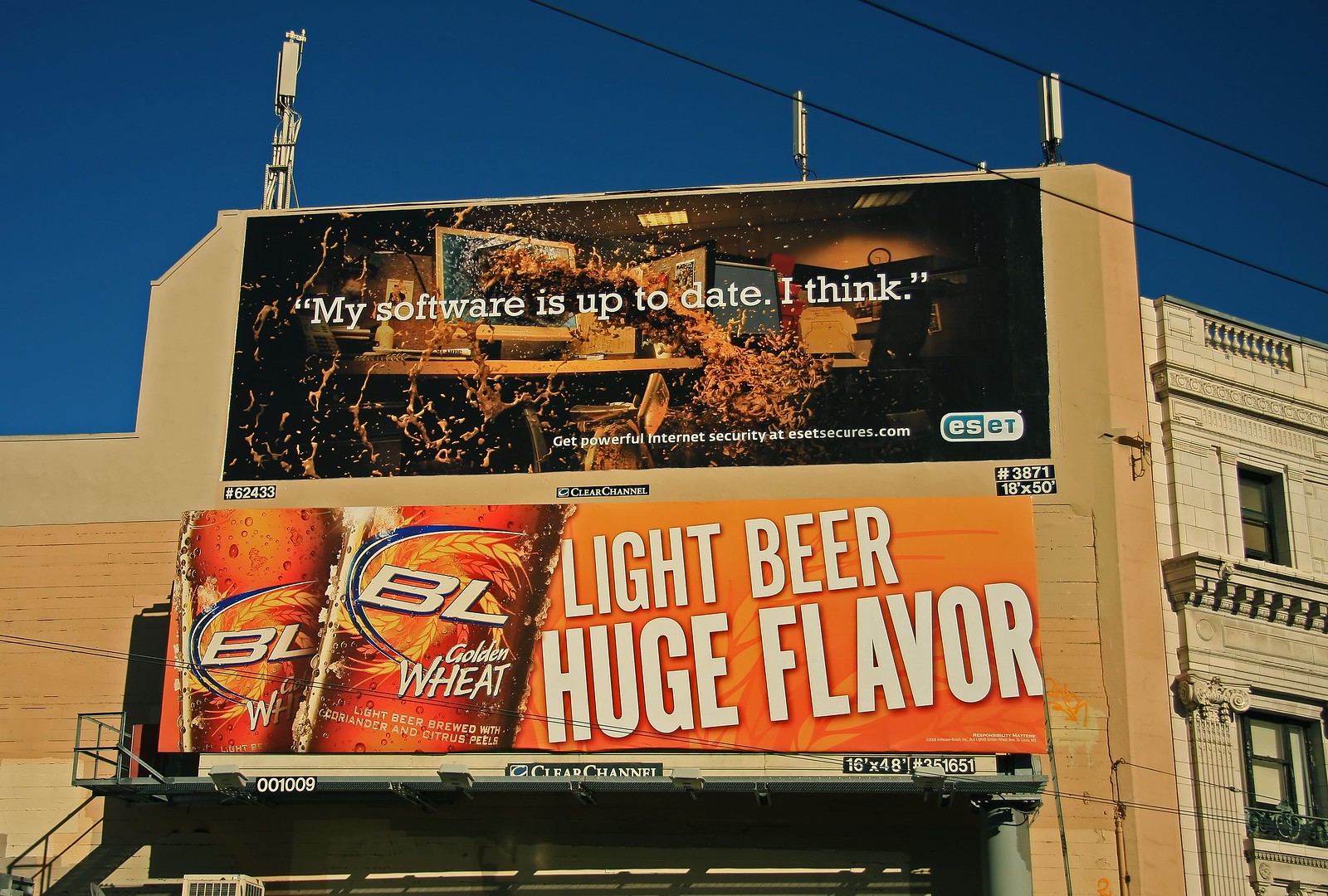The image features two prominent billboard advertisements affixed to the side of a tan building, set against a clear blue sky crisscrossed by black power lines. The upper billboard is rectangular and promotes internet security by ESET. It reads, "My software is up to date, I think," with an accompanying image of an office scene where a virtual explosion appears to be emanating from a computer monitor, spilling disturbing digital elements over the desks. Beneath this, in bold white text, it advises viewers to "Get powerful internet security" and provides a URL to ESETsecures.com, complete with an ESET logo at the bottom right corner. The lower billboard, primarily in shades of orange, advertises Bud Light's "Golden Wheat" beer. It features two glass beer bottles labeled "BL Golden Wheat" and the tagline "Light beer, huge flavor" in large white letters. Additional text indicates that the beer is brewed with coriander and citrus peels. The billboards are sizable, with the top one measuring approximately 18 by 50 feet and the bottom one 16 by 48 feet.